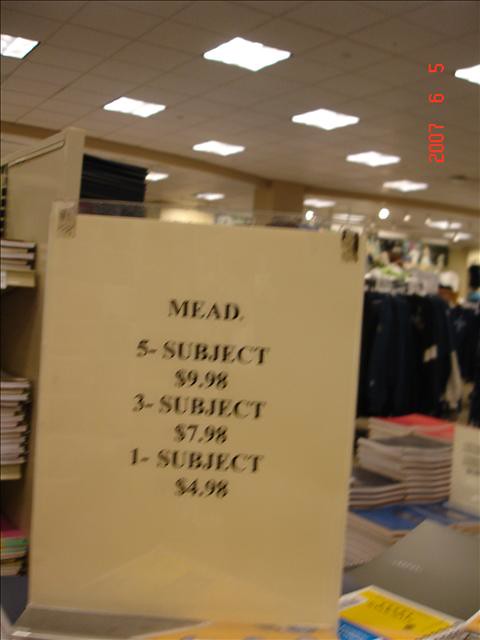The image captures the slightly blurred interior of a retail store, dominated by a prominently displayed sign in a hard plastic frame with a standing base. This white paper sign, seen at a slightly upward angle, details in black lettering: "MEAD" at the top, followed by "5-subject" priced at "$9.98", "3-subject" at "$7.98", and "1-subject" at "$4.98". The overall tone of the image is yellowish, and on the right-hand side, several stacks of spiral notebooks are visible. The background includes shelves filled with books on the left and dark blue clothes hanging on racks. The ceiling features square tile panels with integrated lighting. A vertical red time stamp saying "2007-6-5" is visible in the upper right corner of the frame.